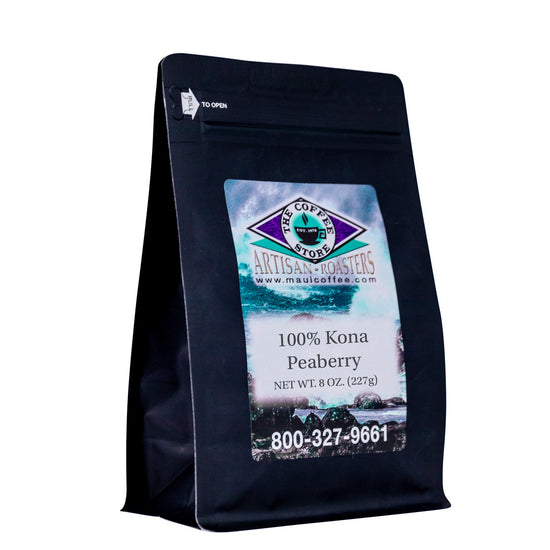This image features a bag of coffee from The Coffee Store, an artisan roaster. The bag is predominantly a dark purple-blue color with a light turquoise background featuring purple triangles on the sides. The top left has an arrow with instructions to “rip open, pull here” for resealing purposes. The bag contains 100% Kona Peaberry coffee with a net weight of 8 ounces (227 grams). The front of the bag prominently displays the website, www.MauiCoffee.com, and a circular logo featuring a steaming coffee cup. Additionally, there's a phone number at the bottom: 1-800-327-9661, adding more detail about the company's contact information. There's also an image of the surf and rocks, suggesting the Hawaiian origin of the coffee.